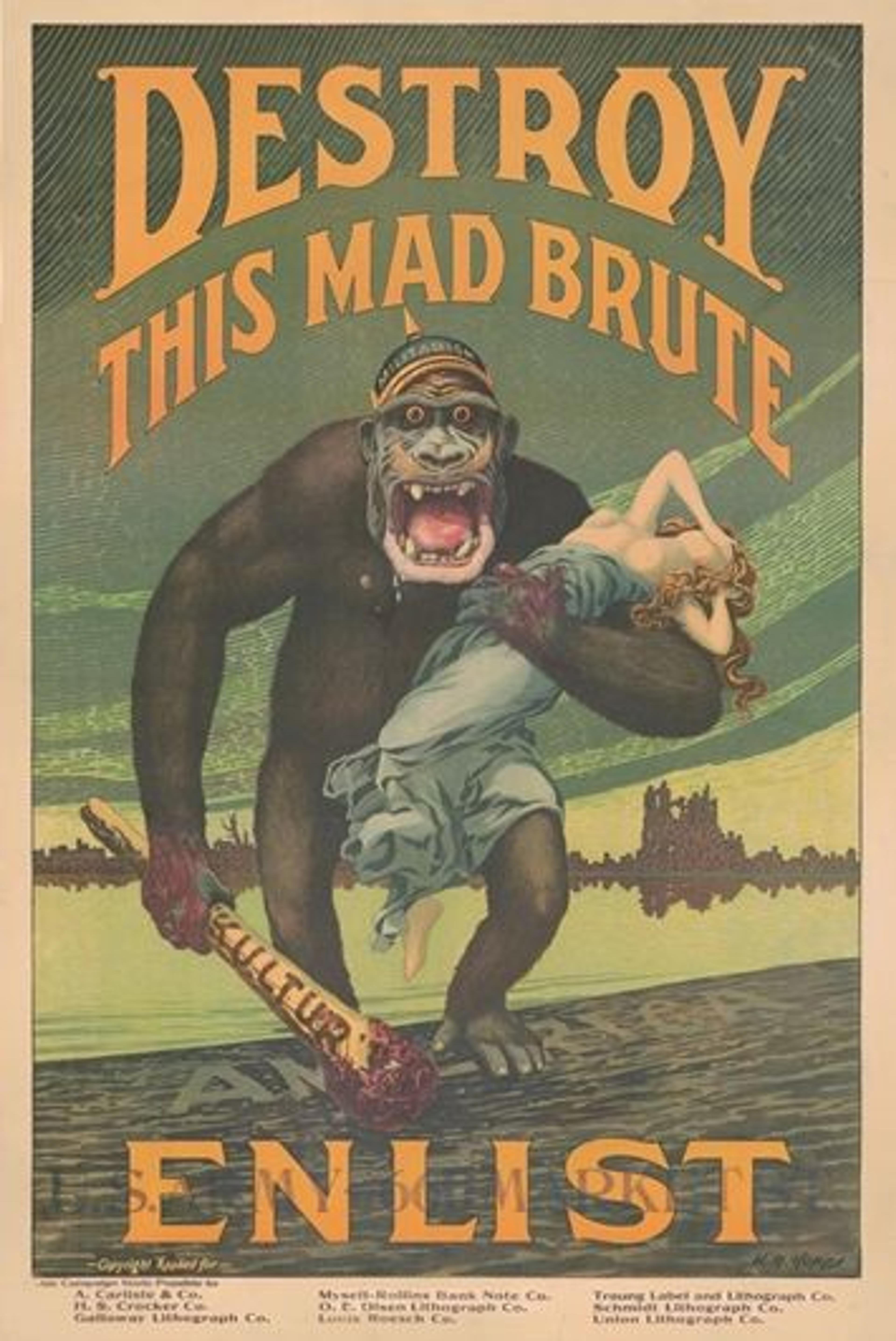This detailed description of an old, promotional military poster captures a scene with a fierce, large gorilla wearing a pointed Kaiser-style cap, with some illegible lettering on it. The poster, tall and rectangular, features a light beige border enclosing a vibrant image. The background is light green, prominently displaying the gorilla facing forward with its mouth wide open, conveying an expression of anger or surprise. In its right hand, the gorilla grips a bloody baseball bat labeled "K-U-L-T-U-R." Its left arm holds a swooning or unconscious woman with yellow curly hair, clad in a blue dress that has slipped down to expose her breasts, her arms raised to cover her eyes. Dominating the top of the poster in large, bold, yellow or orange letters is the phrase "Destroy This Mad Brute," while the word "Enlist" appears at the bottom in a similar font. The gorilla stands over a textured, gray area inscribed with "America," set against a light green background. The poster also includes some illegible text at the bottom, likely names or company details.